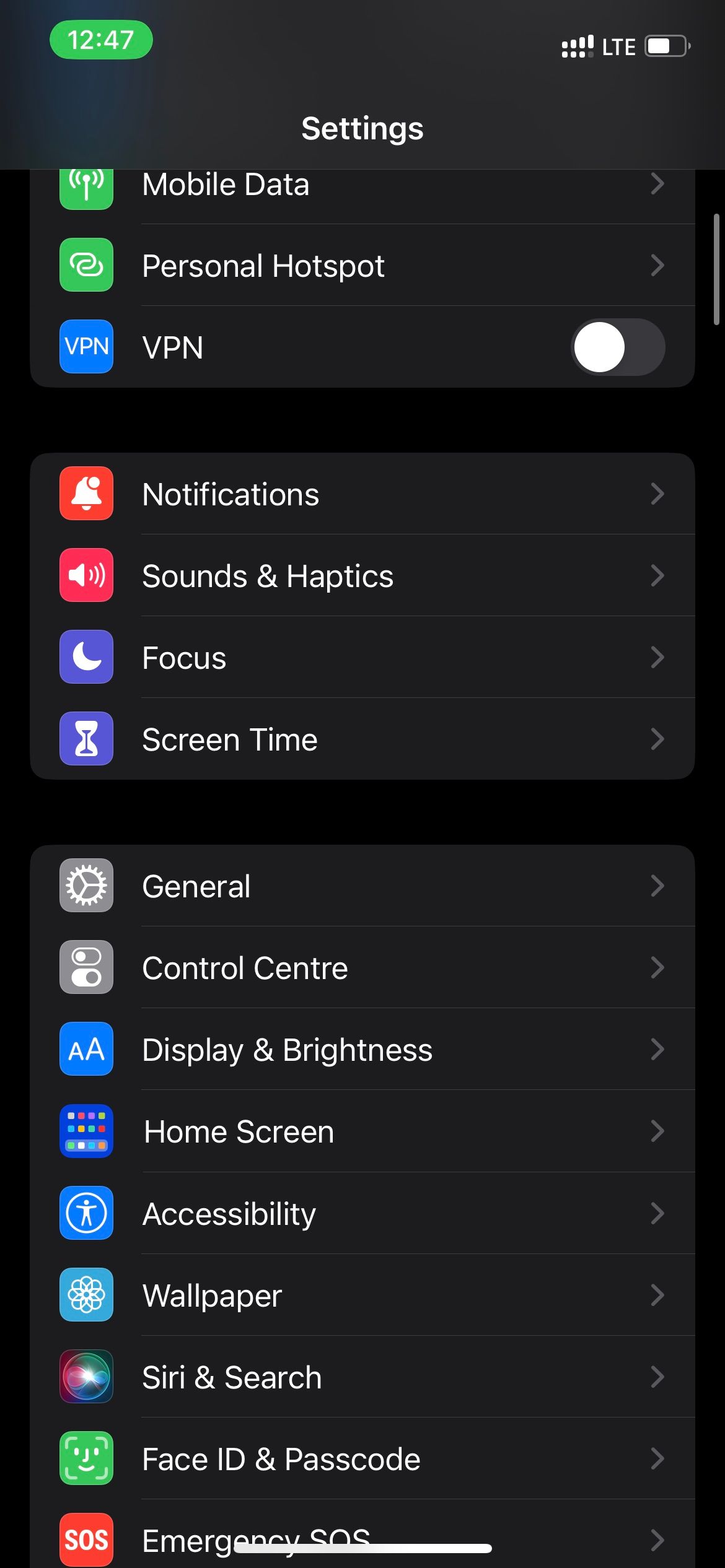A screen capture from an iPhone, displaying the "Settings" menu. At the top of the screen, a green status bar contains white text displaying the time as "12:47," with the indicators for LTE signal and battery status aligned along the right-hand side. Below the status bar, the title "Settings" is prominently displayed in white text. The screen lists various settings options including "Mobile Data," "Personal Hotspot," and "VPN." Further down, options like "Notifications," "Sounds & Haptics," "Focus," and "Screen Time" are visible, followed by additional settings such as "General," "Control Center," "Display & Brightness," "Home Screen," "Accessibility," "Wallpaper," "Siri & Search," "Face ID & Passcode," and "Emergency SOS." Each settings icon is uniquely colored in shades of green, blue, red, purple, gray, yellow, and rainbow colors, enhancing their distinctiveness. At the very bottom of the screen, a small horizontal bar is visible, serving as the navigation handle for toggling between different screens.